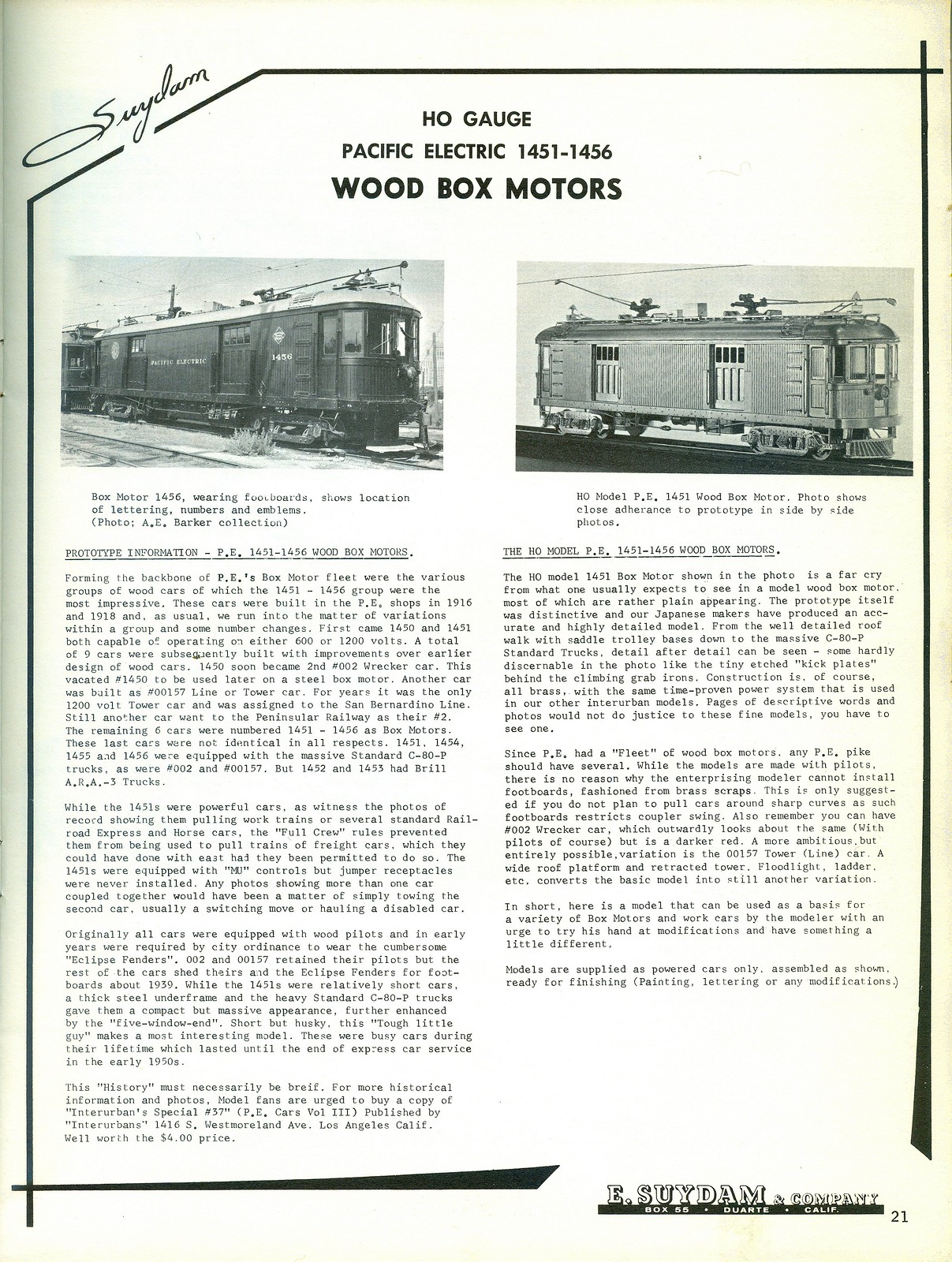The image is a scanned page from a magazine, outlined in a black border. At the top of the page, there are two black-and-white, grainy photographs of vintage train cars. The left photograph features a dark-colored, streetcar-like train with distinctive round windows at the front and two side doors, equipped with wire rail elements on its roof for electric operation. The right photograph depicts a similar train with a dark roof and lighter sides, also showing round windows and two side doors, with the necessary arms for connecting to overhead electric wires.

Above these photographs, there's an underlined title that reads, "H.O. Gauge Pacific Electric 1451-1456 Wood Box Motors." Below the images, the page is filled with dense text, beginning on the left side with the heading: "Prototype Information PE 1451-1456 Wood Box Motors." This section details the history of these train cars, noting that they formed the backbone of Pacific Electric's box motor fleet. Originally built in the PE shops in 1916 and 1918, the 1451-1456 series included variations and renumbered cars, with the initial cars, 1450 and 1451, being capable of operating on either 600 or 1200 volts. In total, nine cars were constructed, each incorporating improvements over earlier wooden designs, with car 1450 eventually becoming the second car numbered 002.